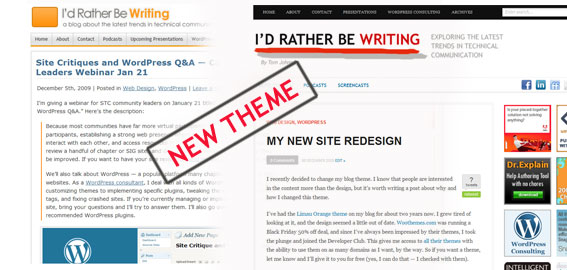The image depicts a webpage from the site "I'd Rather Be Writing." At the top of the page, the title "I'd Rather Be Writing" is presented, with the word "writing" highlighted in orange while the rest of the text is gray. An orange square icon serves as a navigation tool for various sections of the website.

A prominent headline reads, "Site Critiques and WordPress Q&A Leaders Webinar, January 21st," while below, the date "December 5th, 2009" is shown. Nearby, a blue WordPress logo, characterized by a "W" on a white circular background, is visible. 

On the opposite side, the phrase "I'd Rather Be Writing" appears again with a red underline, followed by the tagline, "Exploring the Latest Trends in Technical Communication." 

Centrally located is a black box with red text announcing "New Theme," and beneath it, the subheading "My New Site Redesign" is displayed. 

The page also contains black text interspersed with blue clickable links, alongside social media sharing buttons for Facebook and Indeed, suggesting that users can share the article on these platforms.

Additionally, there's an icon for WordPress Consulting, featuring a "W" and blue text, as well as another icon labeled "Dr. Explain," rendered in orange text.